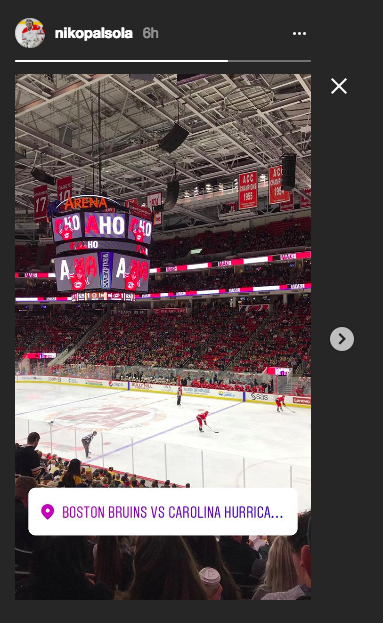This Instagram story captures an intense moment at a hockey game between the Boston Bruins and the Carolina Hurricanes. The background features a vibrant image of an arena packed with enthusiastic fans, most of whom are dressed in red jerseys, eagerly watching the game. 

At the top of the story, text in a clear font reads "Nico Palosola." To the left, there's an inset photo of a player in full hockey gear, poised and ready for action. To the right of this player photo, the text "6 hours" indicates the time left for the story's visibility, followed by three ellipses and a progress bar beneath them. 

Below the top elements, the main image captures the arena's wide expanse, filled with animated spectators. Suspended from the center is a large scoreboard with the text "Arena" and "Aho" in bold letters. The ice below is set for a face-off, with players from both teams—Boston Bruins in their iconic black and gold, and Carolina Hurricanes in their vibrant red—preparing for the play. The referee stands to the side, overseeing the setup with intense focus.

At the bottom of the image, a white rectangular text box displays a caption with a pin mark icon: "Boston Bruins versus Carolina Hurricanes," providing context for the match. To the right side of the image, a circle with a right-pointing arrow indicates there is more content to view in this story. 

This visual composition balances the live-action excitement of the game with informative elements, making it an engaging and comprehensive snapshot for fans following the event on social media.